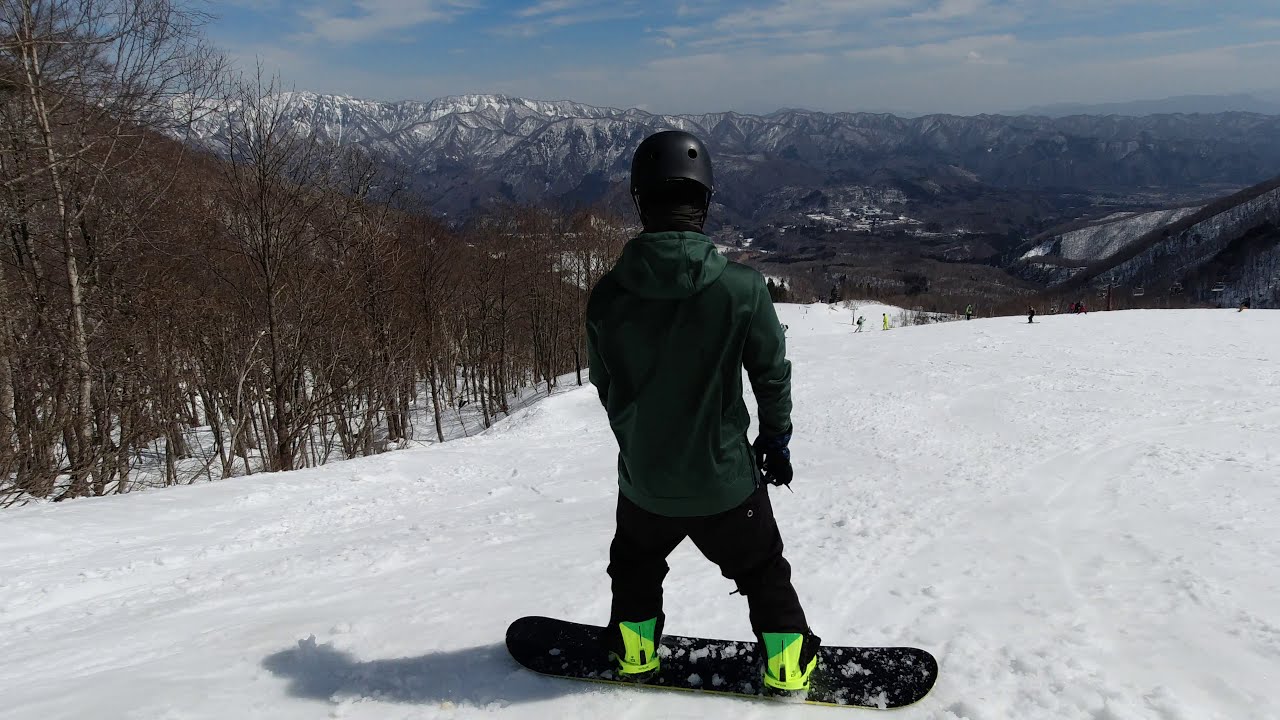A striking photograph captures the serene, snow-covered landscape from the mountain top. In the center of the image stands a solitary snowboarder, his back turned to the camera. Dressed in a green jacket and dark pants with neon green accents, he sports a black helmet and stands poised on a dark-colored snowboard dusted with snow. The snowboarder faces a vast, descending slope that stretches onward, the terrain lined with brown, leafless trees indicative of winter. To the left, the barren deciduous woods form a stark contrast to the icy milieu. Off in the distance, a majestic mountain range looms under a blue sky sporadically adorned with white clouds. Other skiers and snowboarders dot the expansive slope, hinting at the bustling yet tranquil ambiance of the snowy landscape.